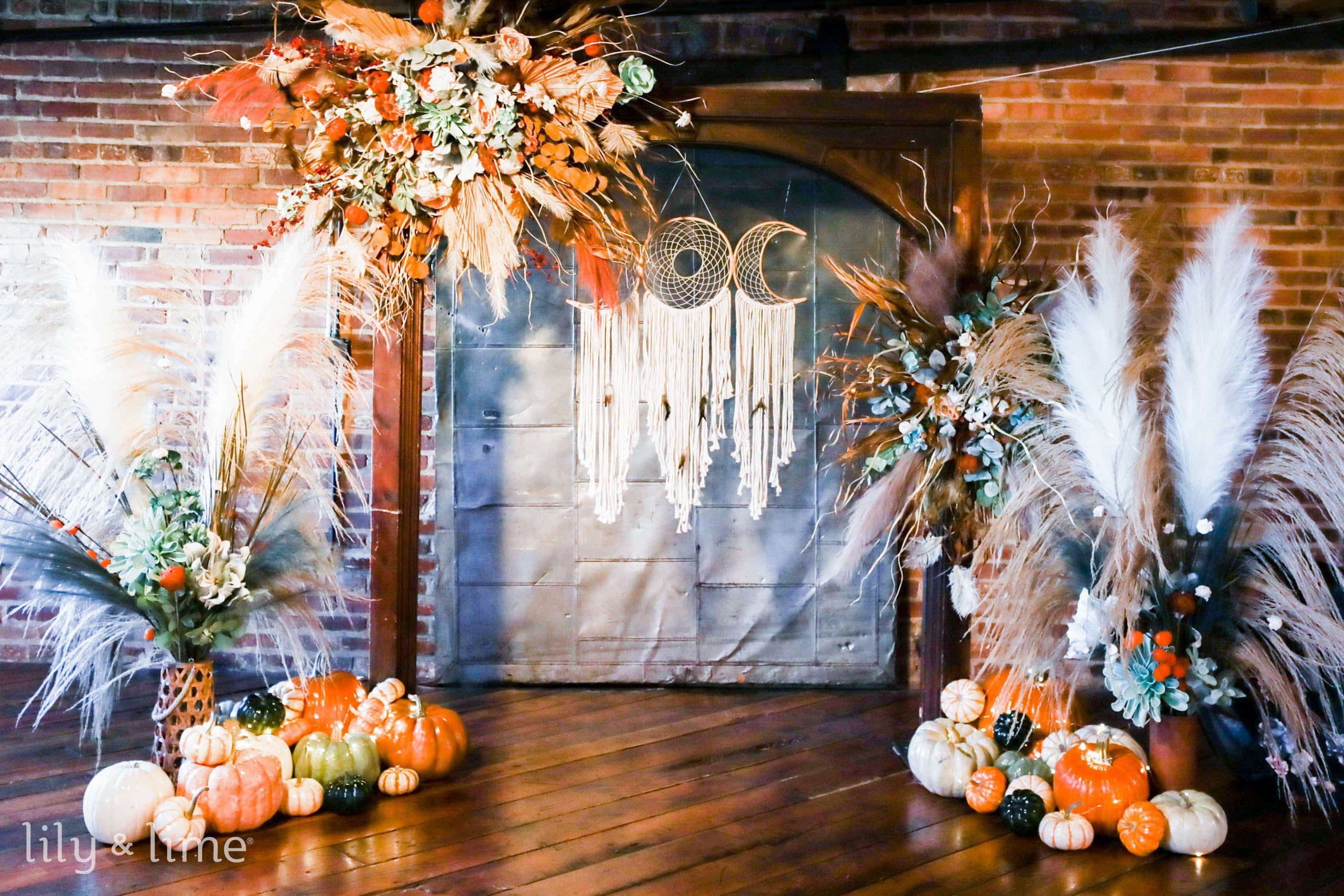This detailed photograph captures an indoor scene centered around a wooden archway, resembling an awning, that frames a metal doorway adorned with a series of dreamcatchers shaped like two crescent moons flanking a central sun. The backdrop features a rich, red brick wall that enhances the rustic, autumnal setting. On the left side of the archway, a large fall decoration hangs, composed of orange, white, and green wildflowers arranged in a cascading bouquet. Beneath it, another bouquet, made of wild weeds and flowers, is nestled in a clay jar surrounded by an assortment of fake pumpkins and gourds, displayed in vibrant fall hues of orange, black, and white. Mirroring this arrangement, the right side also showcases similar decorations, including bright pumpkins, green gourds, and white-tan feather-like plants. The entire scene rests on a wooden floor, exuding a festive and cozy autumn atmosphere.